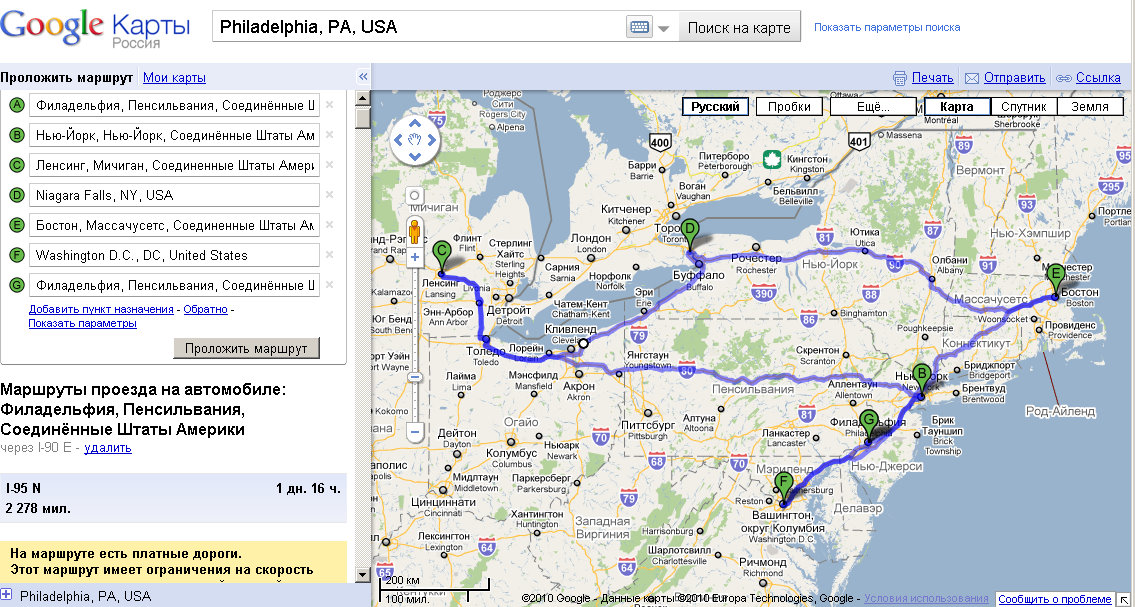The image is a detailed screenshot from Google Maps, displaying a search for directions with Philadelphia, PA, USA typed into the search bar at the top. The map, situated on the right side, prominently features the northeastern United States, encompassing parts of Michigan, Ohio, Pennsylvania, Maryland, New York, Massachusetts, and Connecticut, extending from northern Virginia in the south to as far west as Michigan, but excluding Chicago. The language used in the interface and labels appears to be Russian. 

On the left side of the image, there is a panel listing various routes and directions, identified by green circles labeled A through G. These labels correspond to specific destinations: for instance, C originates north of Lansing, Michigan, and branches to Buffalo, NY, and New York City, while D is marked as Niagara Falls, NY, USA, and F as Washington, DC, USA. The map also shows blue lines indicating the detailed routes between these points, with identifiers in both English and Russian. Specific interstate highways like I-390, I-86, I-81, and I-88 are clearly visible, highlighting the path from multiple locations converging towards key destinations including New York City, Boston, and Philadelphia.